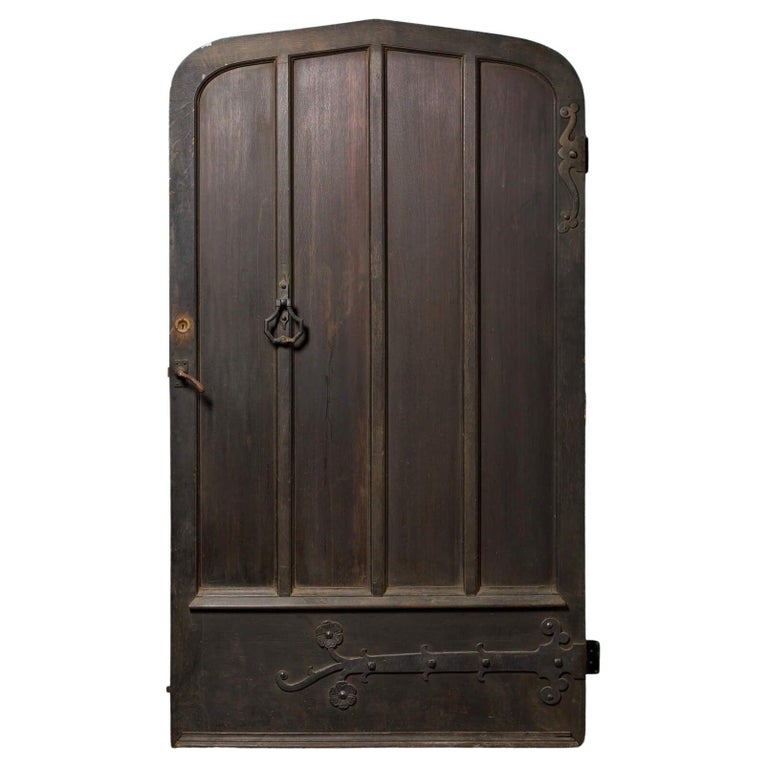This detailed image features a very old, dark brown-black door with a rounded top, almost peaking in the middle. The door's intricate design reveals three vertical lines creating four separate panels. Additionally, there is a large wrought iron panel at the bottom, adorned with two flowers, a branch, and scrollwork. The left side of the door includes a small, skinny handle, a lock, and a keyhole above it. A numbered "2" appears on the upper right corner. A metal knocker, possibly used as a doorbell, hangs on one of the bars. The door's right side features two visible, detailed hinges, with the bottom hinge being particularly ornate with a flowery top. This sturdy door, likely made of wood with some metal elements at the bottom, evokes the feeling of an ancient castle or a very old house. The surrounding part of the image is white, emphasizing the door as the focal point.